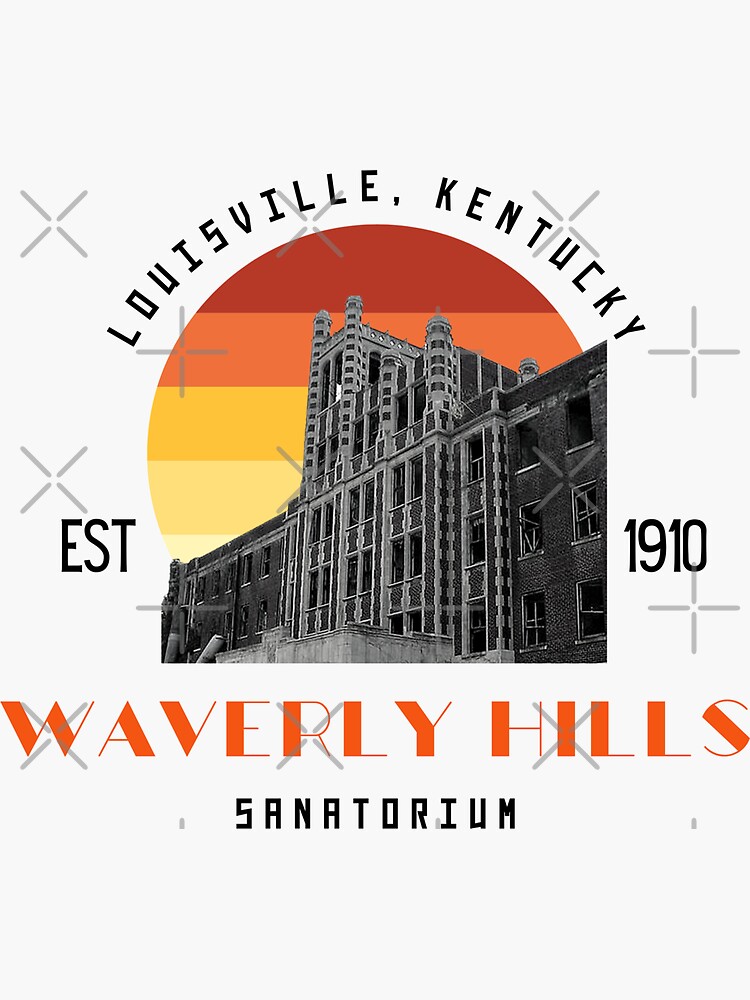This image, set against a white background with a pattern of light gray plus signs or Xs, features a detailed and historic advertisement for Waverly Hills Sanatorium located in Louisville, Kentucky. Centered in portrait orientation, the main focus is a tall, imposing black-and-white photograph of the sanatorium. The building showcases a multi-story structure with a central tower, numerous windows, and a combination of brick facades - including white, gray, and classical red bricks. The windows are notably busted out, giving an eerie, abandoned feel. Above the building, a graphic design element of a gradient sun is superimposed, created from horizontal stripes in shades of red, orange, yellow, and cream, evoking a sense of dawn or sunset. Black text at the top of the image reads "Louisville, Kentucky." Flanking the building image, the text "Established 1910" is displayed, with "EST" on the left and "1910" on the right. Beneath the building, the name "Waverly Hills" is prominently written in red text, followed by "Sanatorium" in smaller black text.